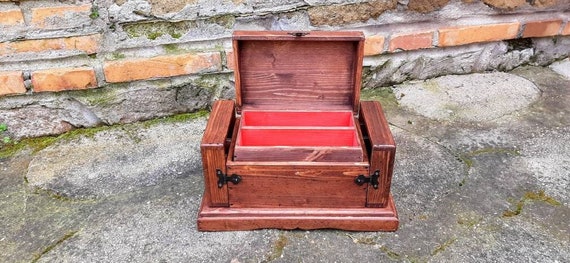The image showcases a serene outdoor setting with the lower section of a stone and brick building in the background, which displays patches of green moss. In the foreground, there is a pavement interspersed with stone elements and speckled with green grass or moss in its cracks. Central to the image is a medium brown wooden box with black metal hinges and two metal clasps, suggesting a sophisticated design. Its lifted lid reveals a plush, red felt-lined interior compartment, segmented into two horizontally oriented, rectangular sections. This well-crafted box, potentially a jewelry or trinket storage box, is nestled against the weathered yet robust background of masonry and verdant growth, hinting at an item of value that contrasts with its rugged surroundings.